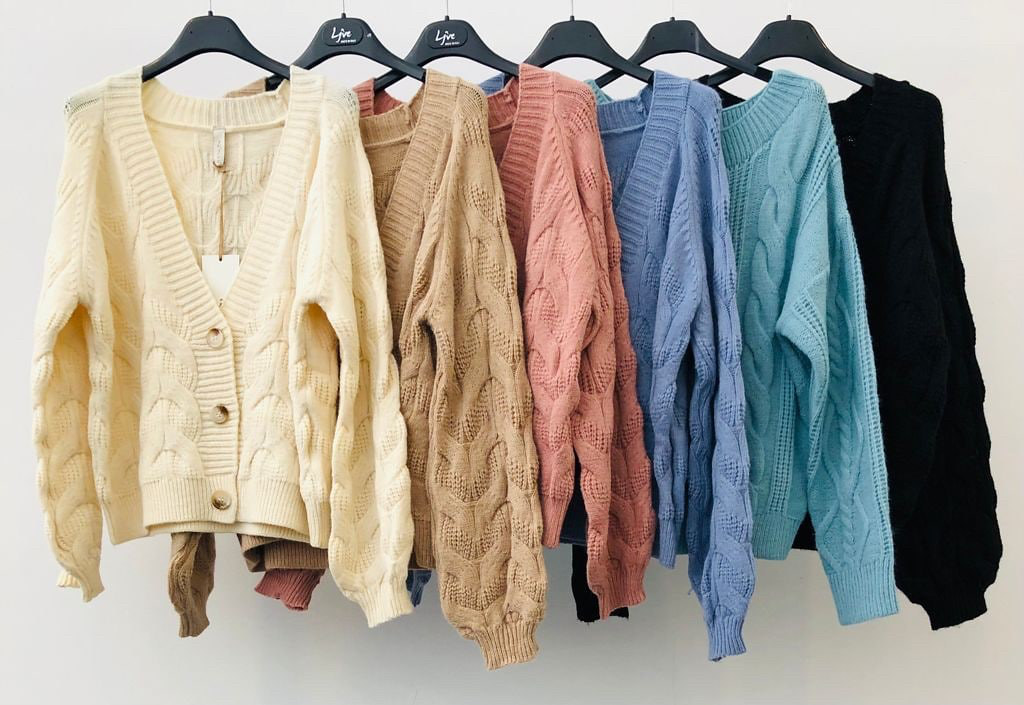This professional photograph features six cardigans neatly arranged on black hangers against a plain white wall background. Each cardigan, identical in design but varying in color, showcases a deep v-neck, long sleeves, three buttons down the front, and a textured woven pattern. Starting from the left, the cardigans are cream, light brown (cappuccino), pink (coral), blue (periwinkle), teal (aqua blue), and black. Notably, the cream and light brown cardigans display a piece of text just below the word "live" or "life." The cream cardigan, which overlays the others in a staggered horizontal arrangement, is visibly new with tags attached by a tan string.